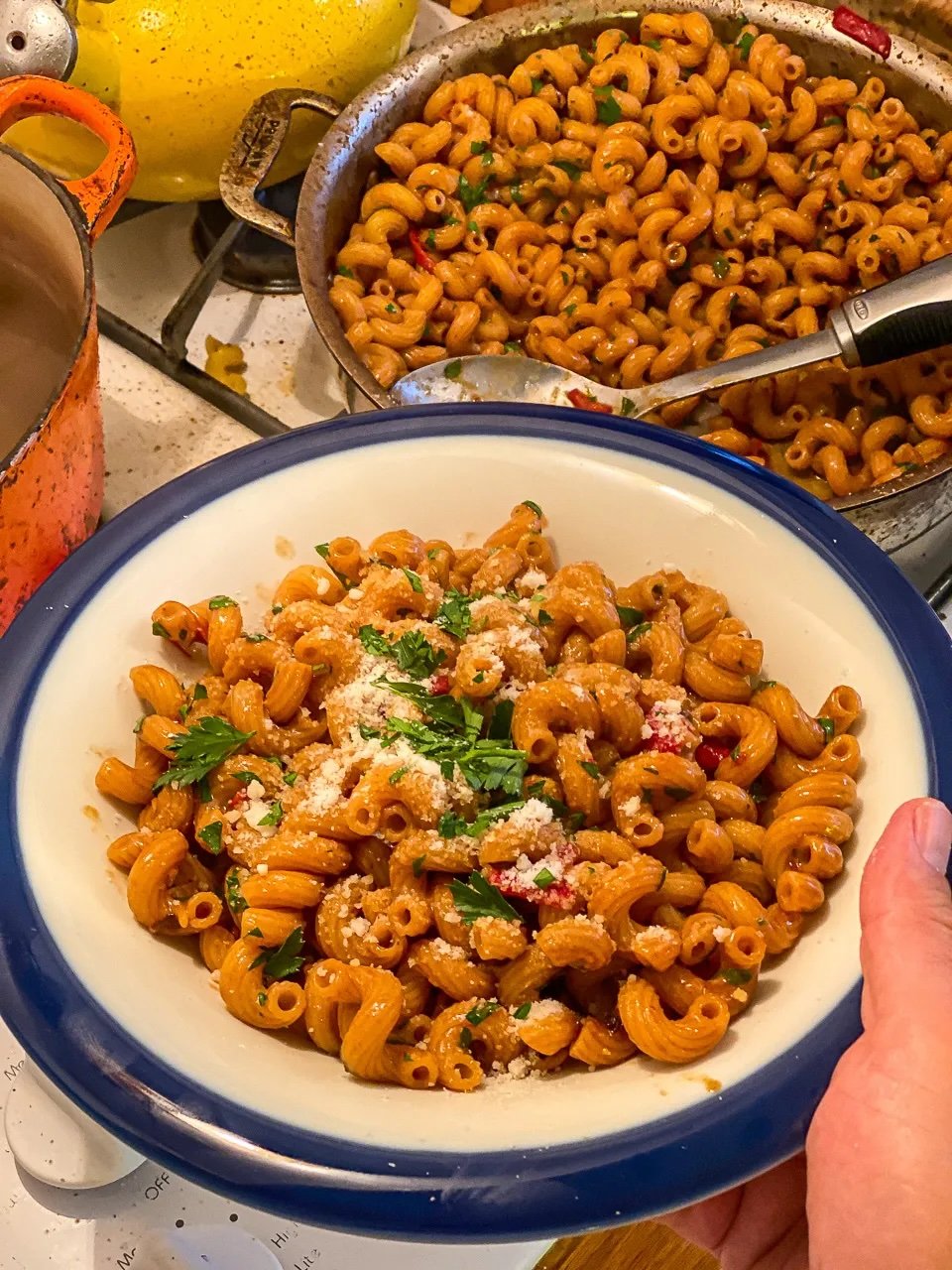In this image, we see a large amount of pasta, specifically small curls of macaroni, coated in a creamy cheese sauce. Scattered throughout the pasta are small green basil leaves, adding a fresh, aromatic touch to the dish. We can also see a generous sprinkling of red, diced tomatoes, providing a vibrant contrast against the golden cheese. A person is holding a plate in their right hand, filled to the brim with this delicious pasta. In the background, there is a very large pan, almost overflowing with the same cheesy pasta, indicating it might be a part of a buffet setup. The setting appears to be a kitchen, as we can spot the knobs of a cooker nearby. The bright, appetizing colors and abundance of food suggest a hearty, home-cooked meal or a gathering.